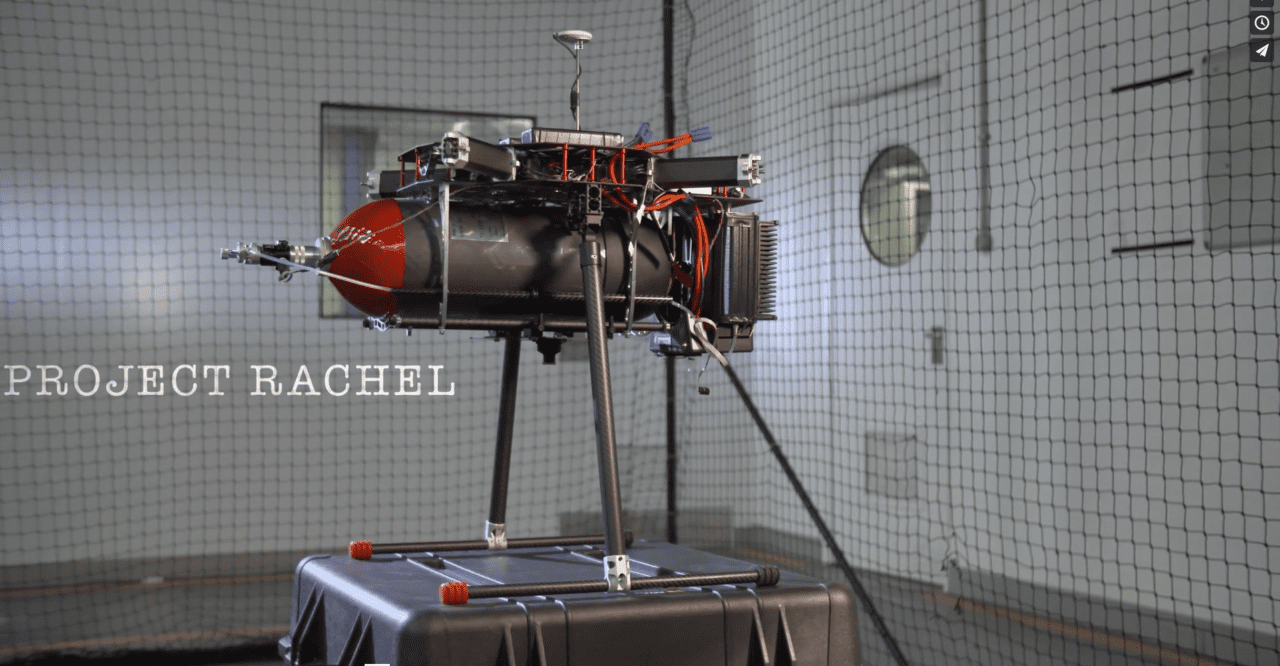The image depicts a detailed close-up of a cylindrical machine, reminiscent of a helium canister or fire extinguisher, situated in a pristine white room. The machine is mounted on a gray square base, resembling a hard metal suitcase or plastic platform, and features two extended arms connecting the base to the device. The machine itself has a red tip and is adorned with various red wires and silver components. The room is enclosed by a black netting that acts like walls on either side of the machine. In the upper right corner of the room, there is a door with a large circular window and text identifying the project as "Project Rachel" written in white font. Additionally, there is a large square window to the left of the door. The setting suggests a scientific or experimental environment.